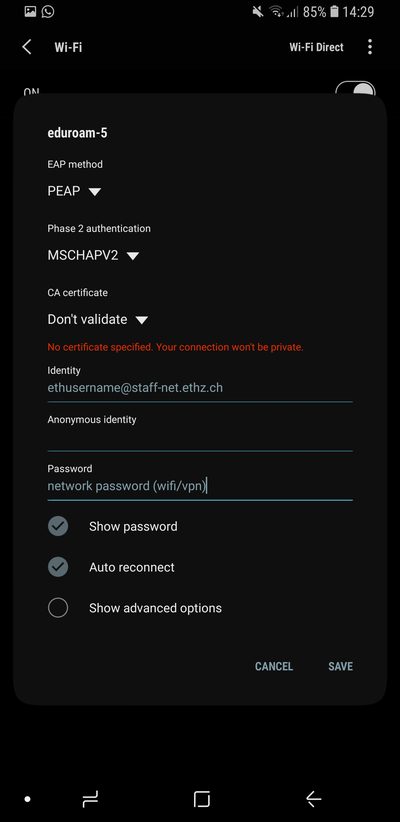The image is a screen capture of a cell phone displaying the Wi-Fi settings screen. The time shown at the top of the screen is 14:29 and the battery level is at 85%. The Wi-Fi is turned on, as indicated by a small sliding button set to the 'On' position. 

Below the Wi-Fi toggle switch, there are several Wi-Fi network options listed, including "eduram" and "eduram-5". For the selected network, detailed settings are displayed:

- **EAP Method:** PEAP
- **Phase 2 Authentication:** MSCHAPV2
- **CA Certificate:** Don't validate (No certificate specified, which means the connection won't be private)
- **Identity:** eth username at staff.net or staff-net.ethz.ch

Additionally, there are various options to tweak the network settings further:

- Password (with a checkbox to show the password)
- Auto Reconnect
- Show Advanced Options
- Cancel and Save buttons are present at the bottom to finalize or discard changes.

The meticulous configuration details suggest that the user is likely customizing settings to connect securely to a specific enterprise or academic network.